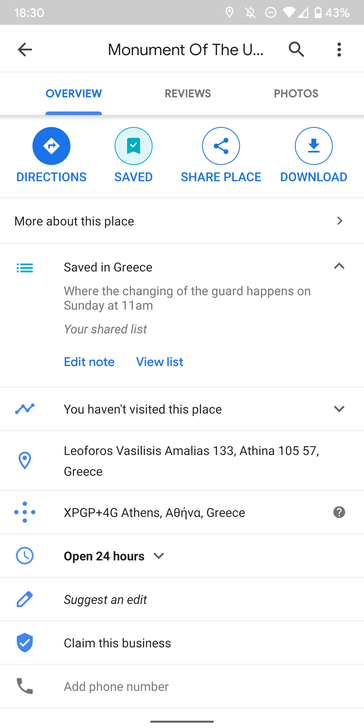The image is a screenshot taken from a smartphone, evidenced by the status icons at the top. Starting from the top right, the screen displays a battery icon showing a 43% charge, adjacent to which is the battery percentage. To the left of the battery icon, there are two signal icons: one depicting the phone signal strength with 2 bars, and the other representing a fully-barred Wi-Fi signal. Moving further left, there's a row of icons including a circle with three dots, a crossed-out bell symbol indicating notifications are silenced, and a location pin icon. On the top left corner, the current time is displayed as 18:30.

Directly below this row of icons lies a search field that reads "monument of the uh". Beneath the search field, there are three tabs labeled "Overview", "Reviews", and "Photos". Following this, there are four more options: "Directions", "Saved", "Share Place", and "Download", each accompanied by its respective icon.

Below these categories, there is a section titled "More about this place", positioned in the middle. Subsequently, there's text indicating the location is "Saved in Greece," with additional details mentioning that the changing of the guard occurs on Sundays at 11 AM. A note suggests that if you haven't visited this place, it is open 24 hours a day, with options to "suggest an edit" or "claim this business". The very bottom of the screenshot features an option to "add phone number".